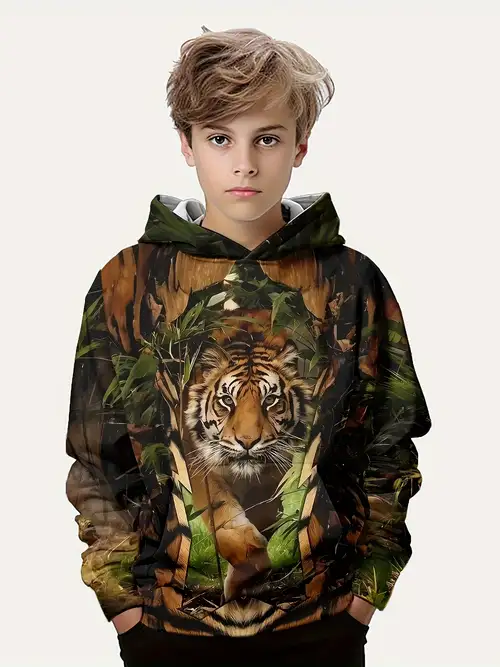In this striking photograph, a young boy stands front and center, looking directly at the camera with a serious expression. His short, slightly messy light brown or blonde hair frames his determined face. He is dressed in a distinctive hoodie that captures the eye with its vivid jungle scene. The most prominent feature of the hoodie is an orange and white Bengal tiger, appearing to emerge through lush, green foliage that covers the chest and torso area. The hoodie itself is a vibrant display of different leaves and plants, with a green hood that is white on the inside. His hands rest casually in the pockets of his dark pants. The entire scene is set against a solid light tan or white background, ensuring that all attention is drawn to the boy and his striking attire.